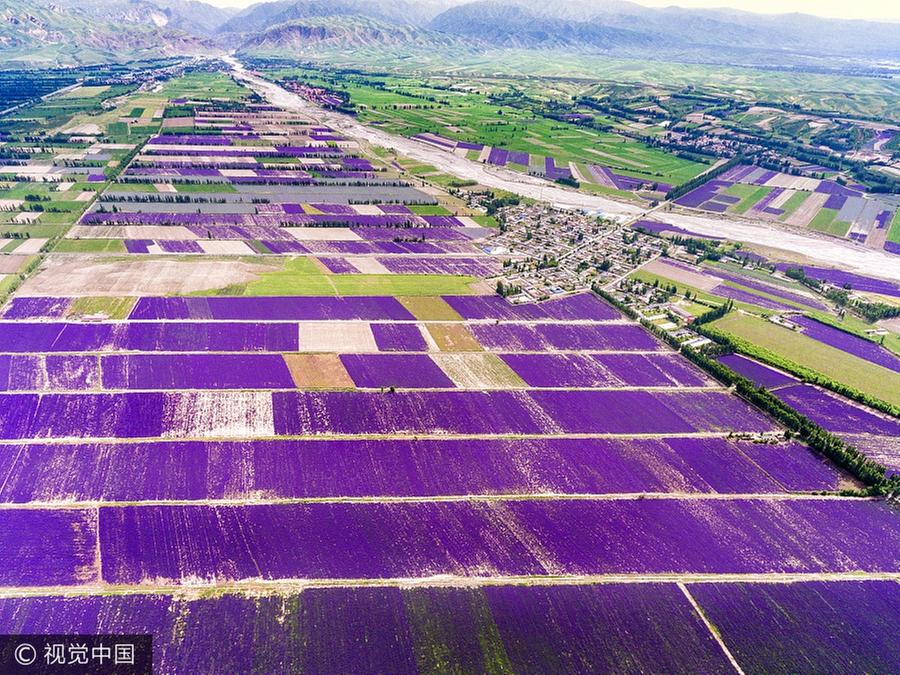This aerial photograph, possibly taken from a drone or helicopter, showcases an expansive farmland landscape characterized by a vibrant patchwork of fields and a sprawling natural backdrop. In the foreground, the primary visual feature is the swath of purple fields, likely blooming with lavender or other types of flowers. These fields are segmented by white lines and interspersed with sparse rectangles of beige and brown, indicating uncultivated or fallow patches.

Further into the landscape, one can observe a mix of green and purple fields, with green fields becoming more prominent towards the peripheries. On the right side of the image, orderly rows of trees separate distinct patches of crops, while additional tree lines and fields appear to the left.

In the upper right corner, a small cluster of houses forms a tiny village, underscoring the rural setting. This area also contains what appears to be a river, adding to the idyllic rural scenery. The entire landscape is framed against a backdrop of tall mountains and canyons, hinting at a mountainous region.

Overall, the image brilliantly captures the contrast between the rich, cultivated farmland and the majestic natural surroundings, providing a detailed and colorful overview of this rural haven.